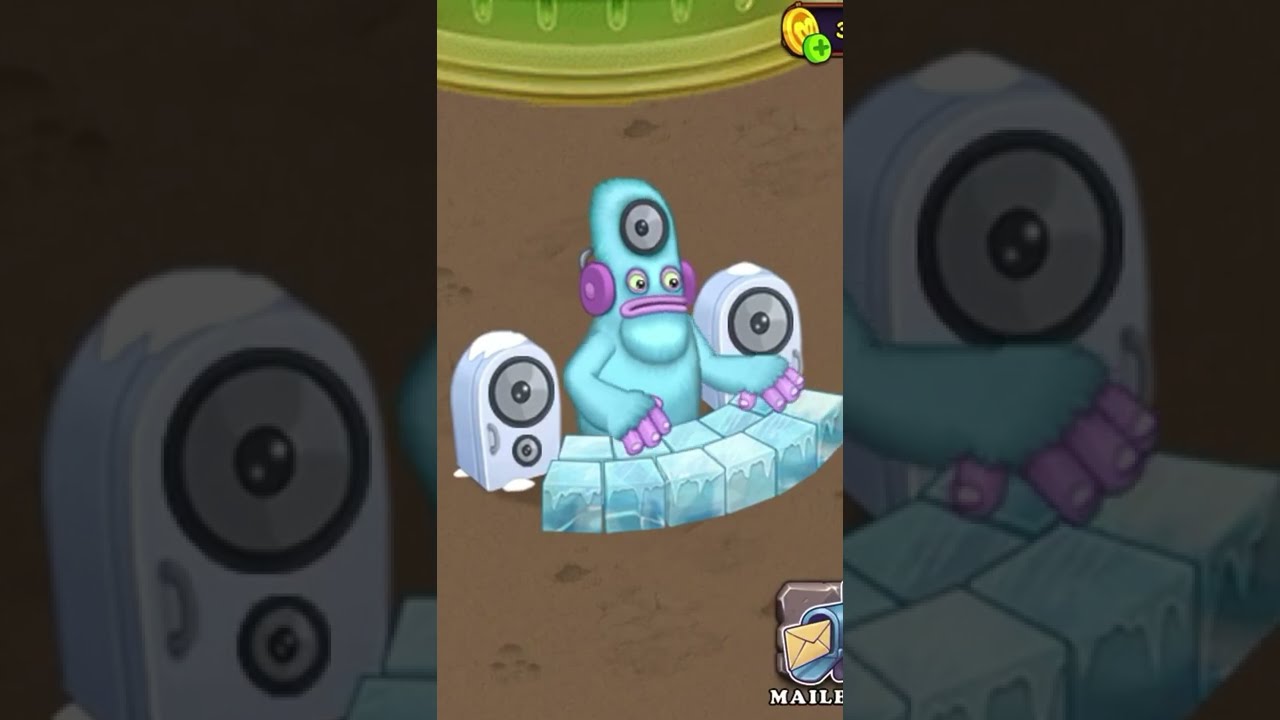The image appears to be a cartoon-style animation or possibly a scene from a video game, featuring a fuzzy, blue, monster-like creature with a rounded head and a circular gray speaker protruding from its forehead. The creature has turquoise fur, purple fingers resembling mini sausages, and purple lips, and it wears matching purple over-the-ear headphones. It stands in a central position, appearing to DJ or play a keyboard created from semicircular-arranged ice blocks or cubes, which resemble the keys of a frozen piano.

On either side of the creature, there are large, white speakers that could also be interpreted as refrigerator-like devices or additional monster figures with handle-like features resembling frowny faces. The background includes a brown floor rug, a greenish baseboard, and a green wallpapered wall. Noteworthy details include a golden coin with a green plus sign located in the upper-right corner of the image and a mailbox in the lower part of the frame. The smaller inset image in the center mirrors the larger scene, highlighting the creature and its DJ setup.